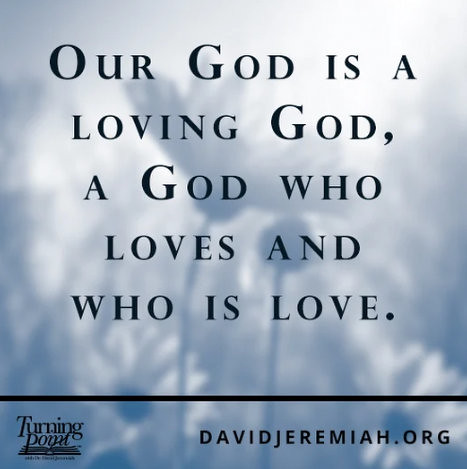The image displays a religious saying on a light gray background adorned with subtly shaded dark gray flowers with stems, and a touch of white at the top. The prominent black text reads, "Our God is a loving God, a God who loves and who is love." At the bottom, a thick dark line stretches across the image. The bottom left corner bears the label "Turning Point," hinting at the source of the quote, while the bottom right corner includes the website "DavidJeremiah.org." The scene is devoid of any human figures or vibrant colors, emphasizing the serene and reflective nature of the message.